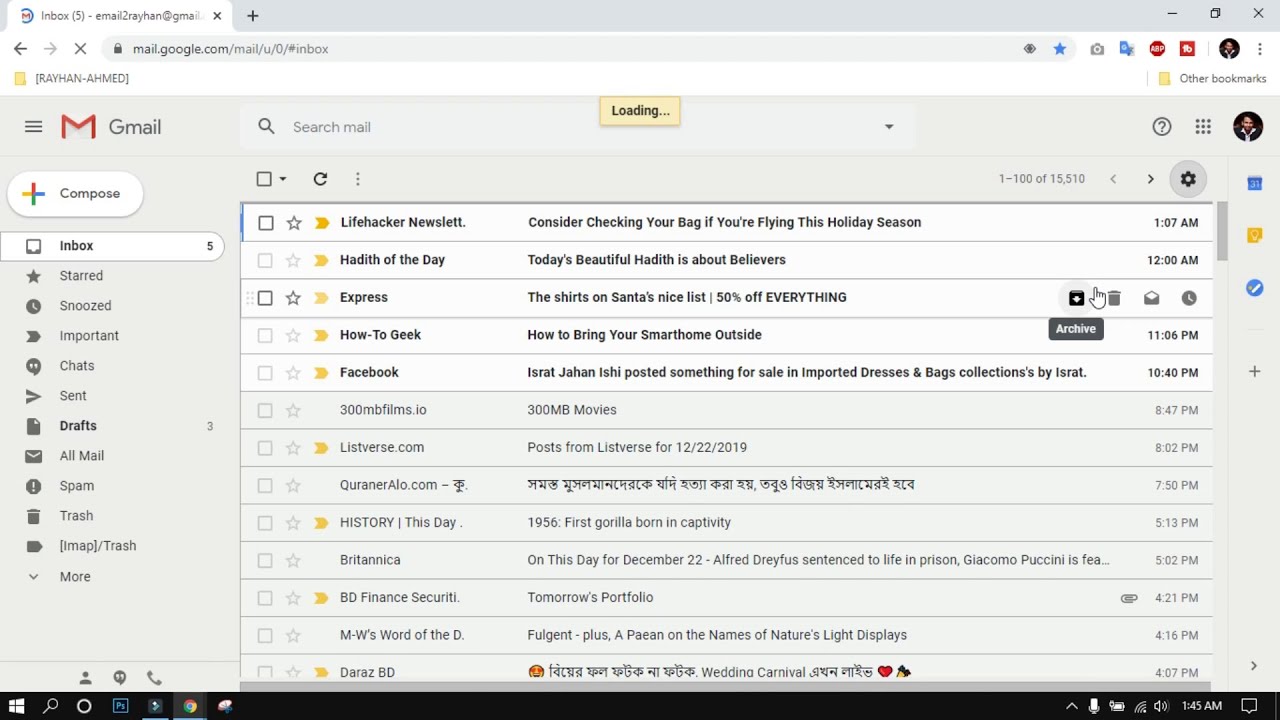This is an image of a Gmail interface, displaying the inbox of a user named Rehan Ahmed. The screenshot captures Gmail mid-loading, with the familiar Gmail logo on the top left, followed by the red, yellow, blue, and green "Compose" button with a plus sign. Down the left sidebar are options such as Inbox, Starred, Snoozed, Important, Chats, Sent, Drafts, All Mail, Spam, Trash, and IMAP/Trash, with some options expanded to show further categories including a total of five unread emails in the Inbox.

The main content area reveals several emails within Rehan’s inbox. Among them are:

1. **Lifehacker Newsletter** with a headline encouraging readers to check their bags if flying during the holiday season.
2. **"Hottest of the Day"** - A daily newsletter or update.
3. **Express Promotions** - Featuring a sale, "The shirts on Santa's nice list, 50% off everything."
4. **How-To Geek** - An email about bringing your smartphone outside in cold weather.
5. **Facebook Notification** - From an Israt Janam about items for sale.
6. **300 MB Movies** - From 300 MB Films.io, likely offering films for download.
7. **Listverse** - A post scheduled for December 22, 2019.
8. **Coroallo.com** - Featuring what appears to be content in Hindi.
9. **Historical Event Notifications** - Including Britannica’s "On This Day" for December 22, mentioning Alfred Dreyfus and Giacomo Puccini, among other historical facts.
10. **BD Financial Security** - An email titled "Tomorrow’s Portfolio."
11. **MW’s Word of the Day** - Featuring the word "Fall Joint."
12. **Nature’s Light Displays** - From a page about the names of various light displays in nature.
13. **Daraz BD** - Featuring more content in Hindi.

The interface also shows numerous tiny clickable icons scattered throughout, likely representing various email actions and features.